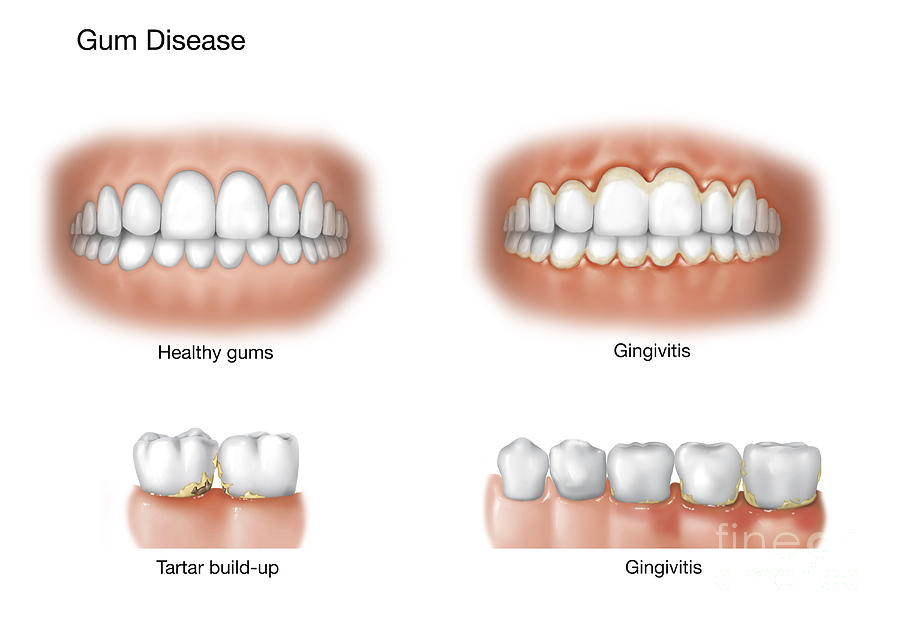This dental poster depicts various stages of gum disease against a plain white background. At the top, the title "Gum Disease" is prominently displayed in black. The first close-up image on the top left shows healthy gums with pink tissue and bright white teeth, labeled "Healthy Gums." Adjacent to it on the top right is an image illustrating "Gingivitis," characterized by inflamed, orange-tinged areas along the gum line. Below, on the bottom left, a close-up of two teeth with visible gray and yellow tartar buildup at the base is labeled "Tartar Buildup." The final image on the bottom right features five teeth exhibiting more severe gingivitis, with irritated, inflamed gums and plaque accumulation around the edges.